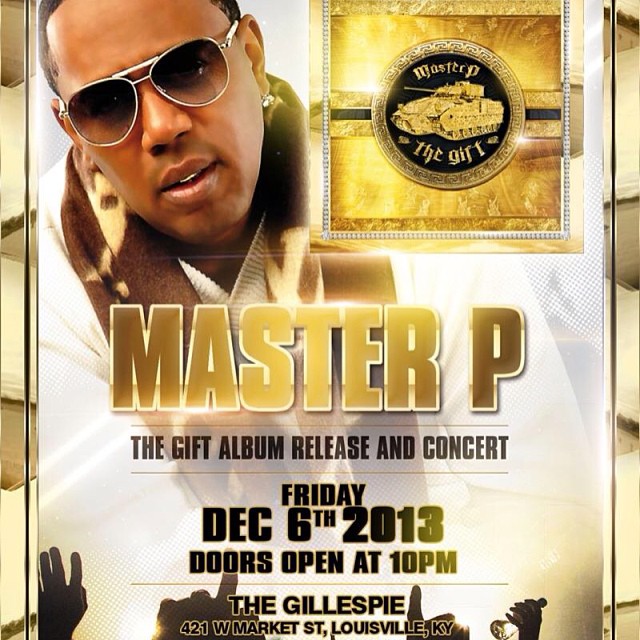This image is a detailed and stylish advertisement for a musical album release and concert by rapper Master P, set to take place on Friday, December 6, 2013, at The Gillespie, 421 West Market Street, Louisville, Kentucky, with doors opening at 10 p.m. The rectangular poster, taller than it is wide, features prominent gold-themed design elements. The left and right sides are adorned with gold bar borders, while the background in the center is primarily white, providing a clean contrast to the vibrant gold accents.

In the top left corner, there is an image of an African-American man, presumably Master P himself, looking towards the viewer. He sports silver aviator sunglasses with gradient brown lenses, a diamond earring in his left ear, and a slightly open mouth revealing the top of his teeth. He is dressed in a white shirt, which melds seamlessly with the white background, and a thick scarf that is brown and tan on the left side, turning green on the right. The scarf adds texture and depth to his attire. 

Dominating the top center of the poster, large, gleaming gold letters spell out "Master P," with a bright white outline, making the name pop against the background. Directly below it, in bold black text, it reads, "The Gift Album Release and Concert," followed by a series of thin pinstripes and essential event details in black print.

In the top right corner, there is a gold-outlined square featuring a diamond-beaded border. The square has a gold background with a central gold circle that houses a black field. Inside this circle is an intricately designed gold tank facing left, with Master P's name above it and "The Gift" written beneath, signifying the album title. This posh and meticulously crafted poster captures both the grandeur and the specifics of the event, promising an unforgettable night.